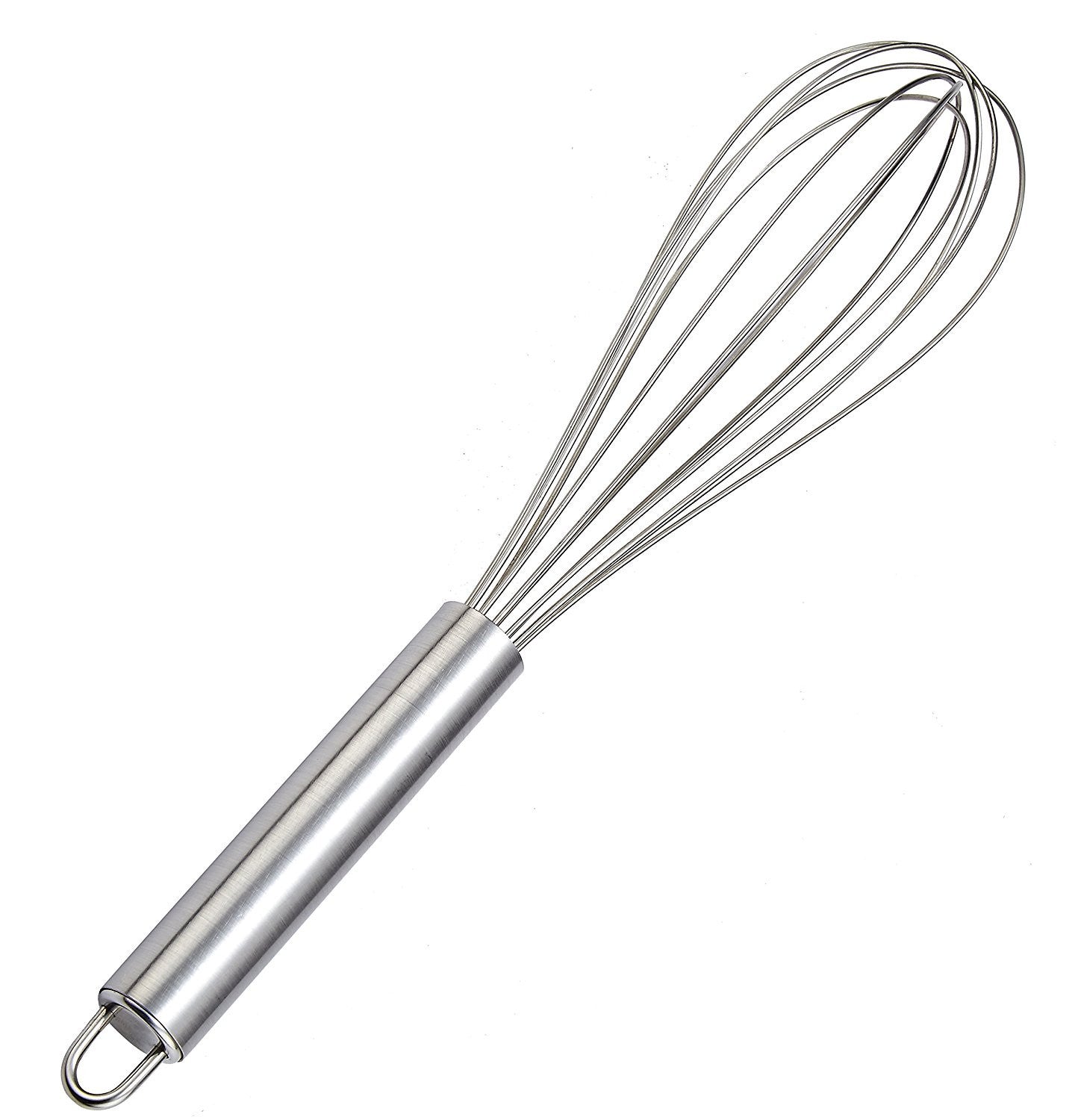The image showcases a stainless steel whisk, featuring a sleek and smooth cylindrical handle that is likely 4 inches in length. At the end of the handle is a sturdy u-shaped hook, ideal for hanging on a hook or utensil carrier. The whisk is crafted entirely from stainless steel, making it easy to clean. Emerging from one end of the handle, possibly around ten stainless steel tines loop over and cross through each other, forming the classic rounded shape ideal for whipping cream, eggs, or mixing liquids and soups. The image focuses solely on the whisk, with no background elements to distract from its design.